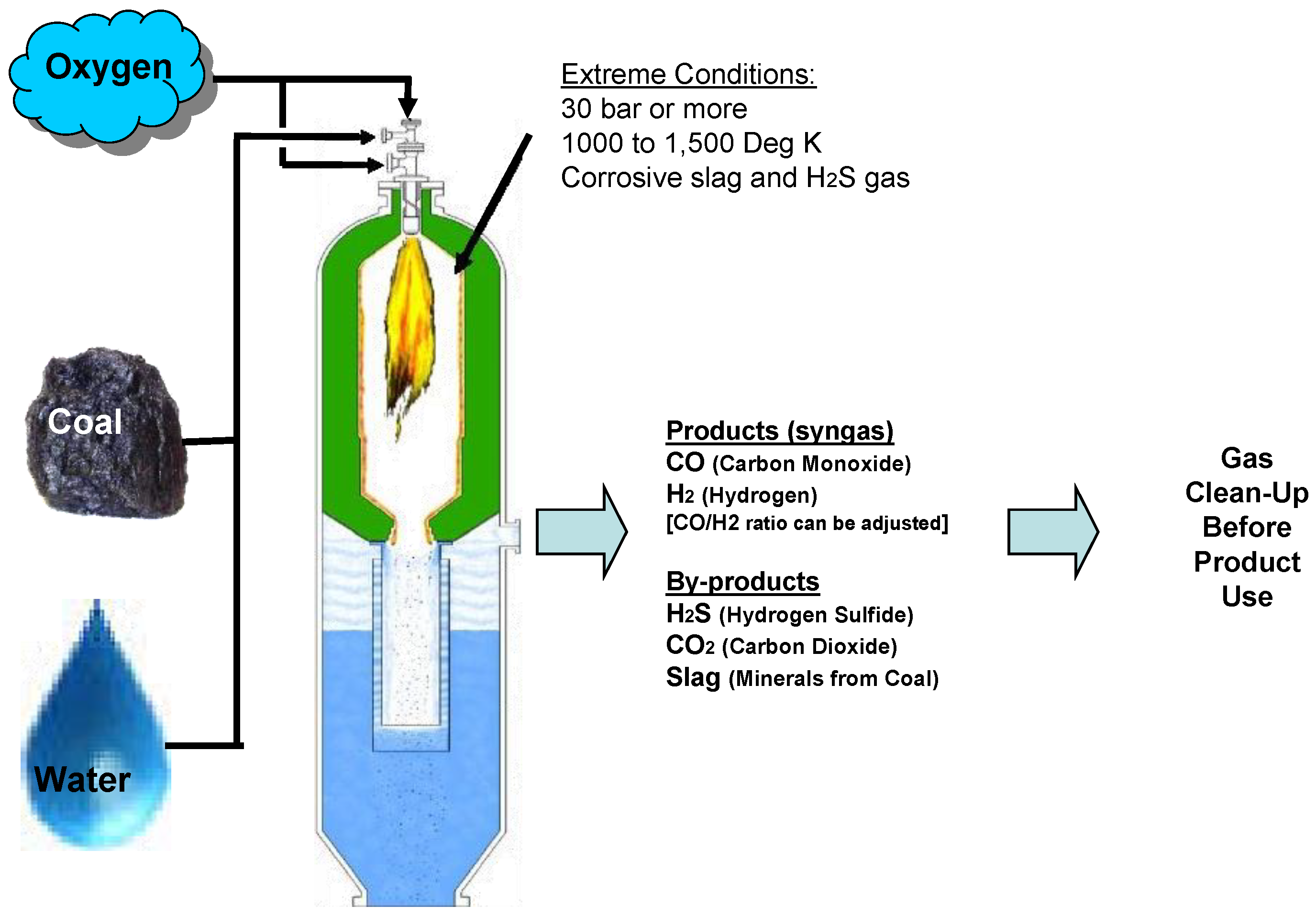The image is a detailed schematic illustrating the various stages and components involved in the process of coal cleaning and byproduct management. Central to the diagram is a test tube-like container that depicts extreme processing conditions, with text indicating pressures of 30 bar or more and temperatures ranging from 1000 to 1500 degrees Kelvin, along with corrosive slag and H₂S gas. The top of the tube features a green section with a yellow flame icon, followed by layers of light blue and slightly darker blue beneath it.

To the left of the tube, three symbols are depicted: a blue bubble labeled "Oxygen," a piece of black rock representing "Coal," and a turquoise water droplet marked "Water." Black arrows point from these symbols toward the central container, indicating the flow of materials into the system. The text next to the tube underscores the severe conditions inside, including the high temperatures and pressures.

On the right side, the schematic details the outcomes of the coal cleaning process, highlighting "Products" such as syngas and "Byproducts" including slag and hydrogen sulfide. An arrow points to a section marked "Gas cleanup before product use," indicating a final purification step before the products are utilized. The overall style of the diagram clearly categorizes and directs attention to each component and stage within the coal cleaning process.